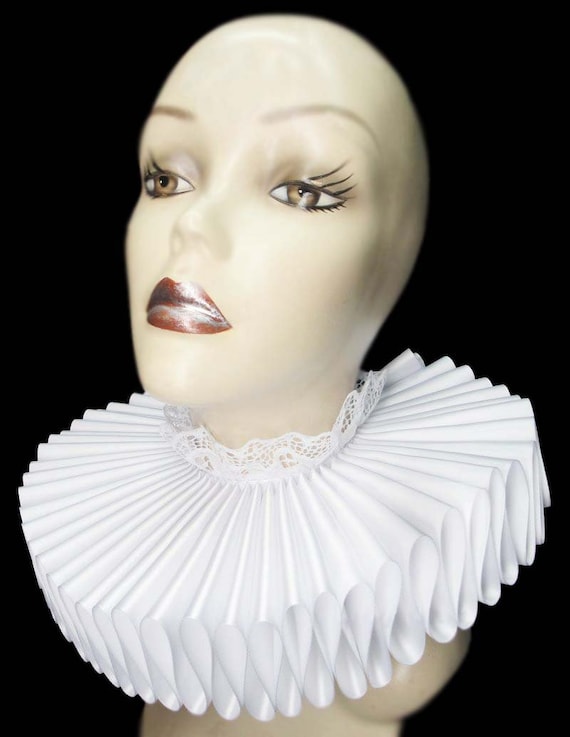In the image, there is a detailed porcelain or ceramic figurine of a woman's head and neck. The figure features an Elizabethan-style accordion collar around its neck, intricately ruffled with layers of white lace extending up the neck. The head is completely bald, accentuating its stark, striking appearance. It has a very pale, almost porcelain skin tone and wears dark wine-colored lipstick that stands out vividly against the pale face. The eyebrows are light, almost barely there, drawn in long, arching lines. The eyes are wide and brown with three stark, drawn-on eyelashes on both the top and bottom lids, giving it a whimsical yet eerie quality. Set against a completely black background, this figurine's detailed features—including the highly ruffled lace collar and finely painted facial features—create a striking contrast, making it appear almost 3D.